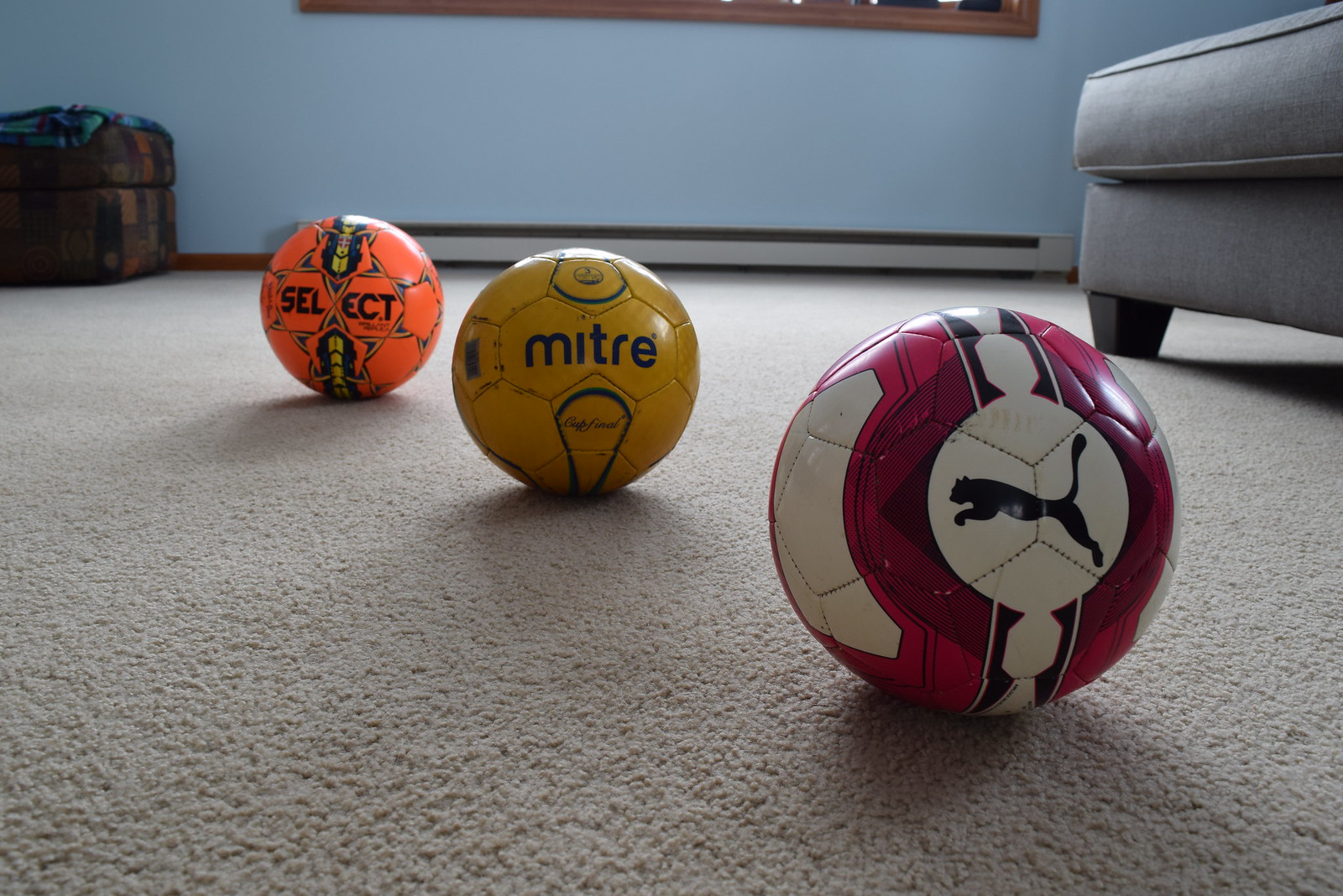The image showcases three soccer balls arranged diagonally in a well-lit living room. The foreground reveals the closest ball, which is burgundy, pink, and white, adorned with the Puma logo. Positioned behind it to the left is a yellow and black ball labeled Miter. The furthest ball, an orange one inscribed with Select, appears to have a distinctive pattern resembling a spiral around its center. The balls rest on a white, rug-like carpet, with a gray ottoman and a plaid storage ottoman draped with a blanket positioned nearby. Natural light streams through a window, partially visible with its trim and an air conditioning unit, casting a warm glow across the scene. A couch is also discernible in the background, adding to the cozy, homely ambiance of the room.